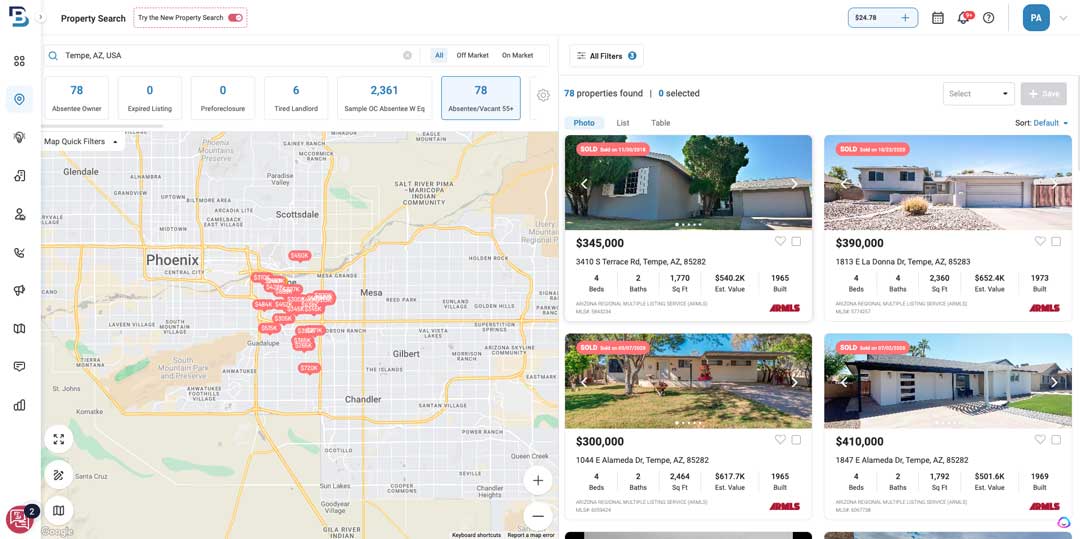In this property search listing for Tampa, Arizona, USA, the interface provides various options to customize search results at the top, including toggles for "all off-market" and "on-market" properties, along with other filtering choices just below. A map dominates the left side, marked with red circles indicating property locations across several cities such as Glendale, Mesa, Phoenix, Scottsdale, Gilbert, and Chandler. To the right of the map, four property listings are displayed. The first listing is priced at $345,000, followed by the second listing at $390,000. Below these, the third home is listed for $300,000, and the fourth property is priced at $410,000. All four properties are ranch-style homes located in the Tampa, Arizona area, offering potential buyers a clear visual and financial overview of the market.